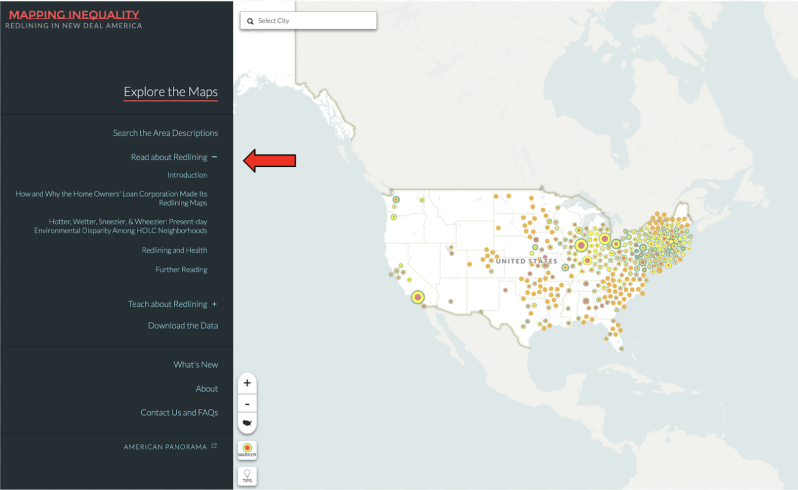This is a detailed and refined caption based on the given voice description:

---

The webpage displays a zoomed-out map of the United States, prominently in white, dotted with numerous pins or markers in varied colors—orange, light green, forest green, yellow-green, and yellow-red combinations. The majority of these pins are concentrated along the eastern coast, with notable clusters in California, the Midwest, and the central regions of the United States. 

At the top left of the map, a search bar featuring a black magnifying glass icon includes the placeholder text "Select City" in gray. To the right, bold black text reads "Mapping Inequality," with the subtitle "Redlining in New Deal America" in gray. Adjacent to this heading, a red arrow points leftward towards an informational list.

The list begins with "Explore the Maps" underlined in red, followed by several sections in light blue text:

1. "Search the Area Descriptions"
2. "Read About Redlining" (accompanied by a rightward arrow signifying a dropdown)
3. "Introduction"
4. "How and Why the Homeowner's Loan Corporation Made Its Redlining Maps"
5. "Hotter, Wetter, Sneezier, and Wheezier: Present-Day Environmental Disparity Among HOLC Neighborhoods"
6. "Redlining and Health"
7. "Further Reading"
8. "Teach About Redlining" (indicated by a plus symbol)
9. "Download Data"

Further down, there's a space followed by sections titled "What's New," "Contact Us," "FAQs," and "American Panorama," the latter being highlighted with a square and an outward-pointing arrow suggesting an expandable section for sharing data.

To the right of the list, navigation controls include an oval with plus and minus signs for zooming in and out of the map and an icon of the United States in black. Additionally, a square icon features green, yellow, and red dots in the center, likely for toggling certain map layers, though the accompanying labels are too small to read. Another icon with small pin marks is also present but similarly challenging to decipher.